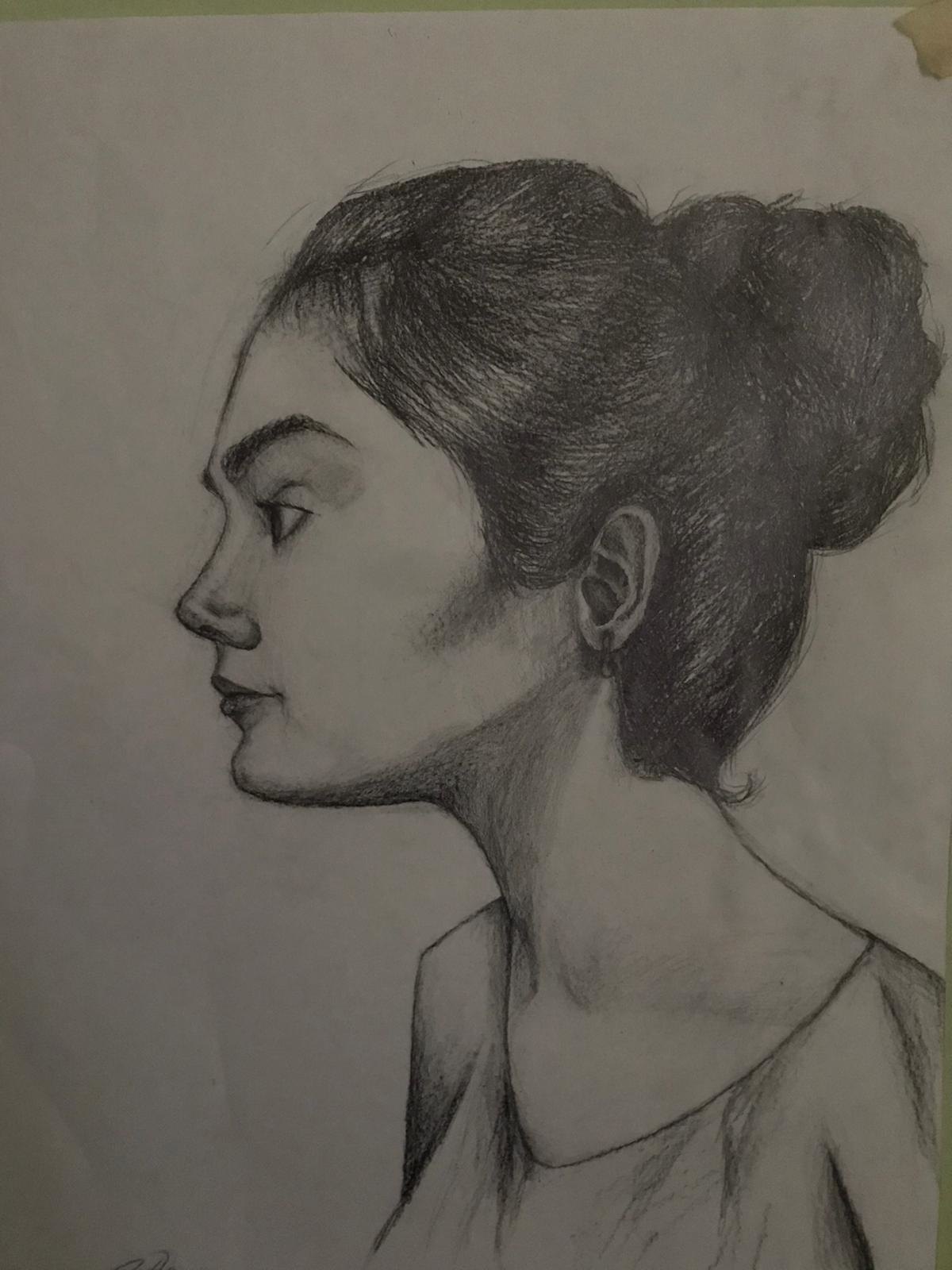This detailed pencil sketch on white paper showcases the profile of a woman with her hair neatly tied up in a dark bun, possibly brown or black. A small watermark stain is visible in the top right corner of the paper. The woman has a neutral expression with arched, medium-thickness eyebrows, a straight and slightly pointy nose, and full lips. Her high cheekbones and slightly protruding chin are distinctly rendered. Notably, she wears a dangling earring on her left ear and a v-neck top that could be a blouse, t-shirt, or dress. The careful shading and attention to detail reflect the artist's skill in portraying the subtle contours of her features and the texture of her hair. Additionally, the overall impression suggests she might be of Hispanic, Middle Eastern, or Southern European descent, and her elegant neck adds to her attractive appearance.